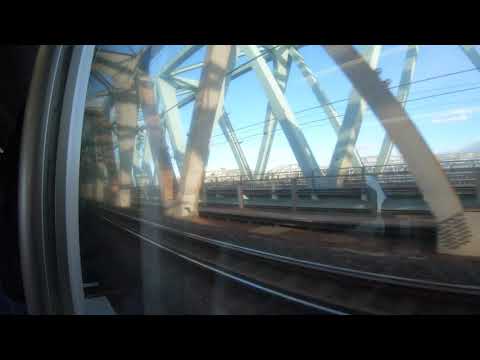This wide rectangular image, bordered at the top and bottom by thick black rectangles, captures a scene from inside a train car, looking out through a window. On the left side of the image, a curved, silver metal bar is visible, possibly part of the train's interior. Reflections can faintly be seen in the window glass. Outside the window, the scene features a train track, which appears to traverse a bridge. The track is brown and silver, stretching across the bottom half of the image. Beyond the tracks, a bridge supported by crisscrossing large silver metal beams dominates the view, with the beams extending in various directions, reminiscent of typical bridge construction. The bright blue sky, dotted with a few white clouds, can be seen through these structural beams, adding contrast to the metallic elements. In the background, there are vague indications of additional structures, possibly hinting at urban buildings. The image sharply depicts the juxtaposition of industrial elements with a serene sky.